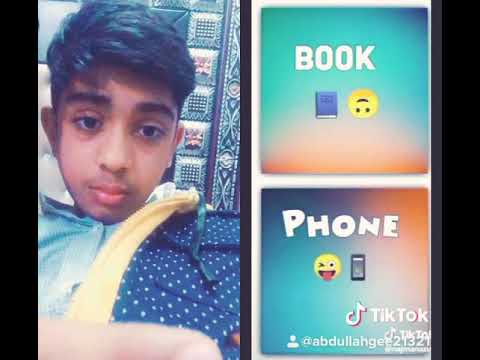The image portrays a teenage boy of Middle Eastern or Indian descent with dark brown skin and short, dark black hair. He is dressed in a navy blue polka-dotted jacket with a yellow zipper and a light blue shirt underneath. The boy, who has thick eyebrows, appears to be taking a selfie, gazing slightly downward at the camera. The photo quality is somewhat grainy. The image is in a split-screen format, with the boy occupying the left side. 

On the right side, there are two square blocks with color gradients ranging from blue to orange. The top square features the word "book" in white font, accompanied by a picture of a book and an upside-down yellow smiley face emoji. The block below showcases the word "phone" in the same white font, alongside a winking smiley face emoji with its tongue sticking out and a cell phone emoji. Below these squares is the TikTok logo and the user’s handle, indicating that this is likely a screenshot from a TikTok video. The background behind the boy is indistinct and could be either indoors or outdoors, with various designs and stands visible.